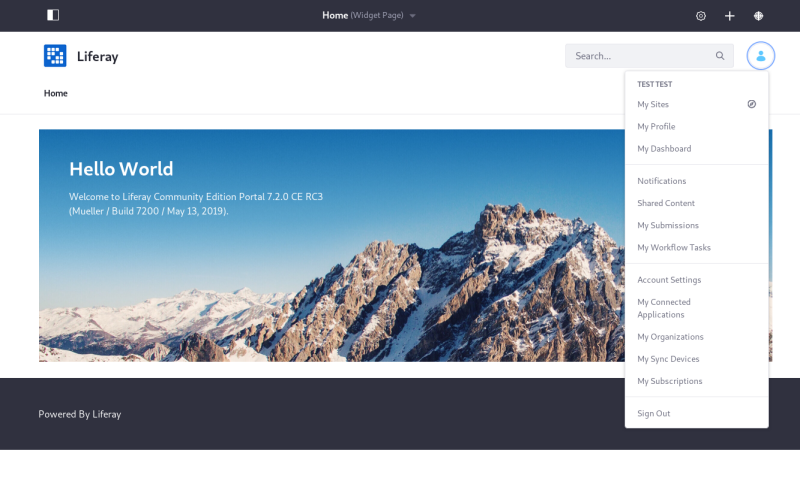A screenshot of a website is displayed. The top banner of the page is thin and black, featuring the word "Home" in white text at the center. Adjacent to "Home," within parentheses, "Widget Page" is written in white print, accompanied by a down arrow symbol.

Beneath this banner, there is a wide white section at the top. Positioned within this area, a blue square containing small white dots encapsulates a centered brand logo "Liferay" written as a single word in black, with a capital 'L'.

To the right of the Liferay logo, a search bar is apparent, labeled "Search" and iconized by a magnifying glass symbol. Adjacent to the search bar is a blue circle, featuring an icon of a person, indicating access to user-related features. When clicked, this reveals a drop-down menu with multiple options: Test Test, My Site, My Profile, My Dashboard, Notifications, Shared Content, My Submissions, My Workflow Tasks, Account Settings, My Connected Applications, My Organizations, My Sync Devices, My Subscriptions, and Sign Out.

Below the white section, the main content appears, dominated by an expansive image capturing an outdoor scene of sky and snow-covered mountains. Overlaying this scenic view, bold white text declares "Hello World". Below, a smaller white text welcomes users to "Liferay Community Edition Portal 7.2.0 CE GA3".

At the bottom of the page, a wider black footer section specifies "Powered by Liferay" in black print, reaffirming the platform's branding.